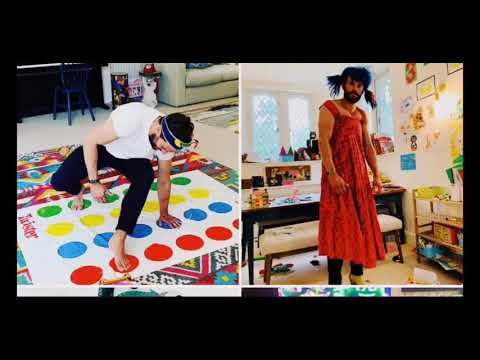The composite image showcases two side-by-side photographs of a man in different settings. In the left photograph, the man is engaged in a game of Twister, dressed in a white shirt and black pants, and is barefoot. The Twister mat is laid out on a brightly colored carpet with geometric patterns. The room features a beige couch, a piano with a blue chair in front of it, and a richly decorated interior. The man has one foot on a red circle, a hand on a blue circle, and the other foot on a green circle.

In the right photograph, the same man is dressed in a long red dress with his dark brown hair styled in pigtails. He stands in what appears to be a children's playroom, facing the camera. The room has white walls adorned with various pictures and artwork. Behind him is a shelf cluttered with objects, a white bench, and a black table placed in front of a window. The floor is covered in light-colored carpet. Additional elements like a chair or stool are also visible, enhancing the playful atmosphere of the room.